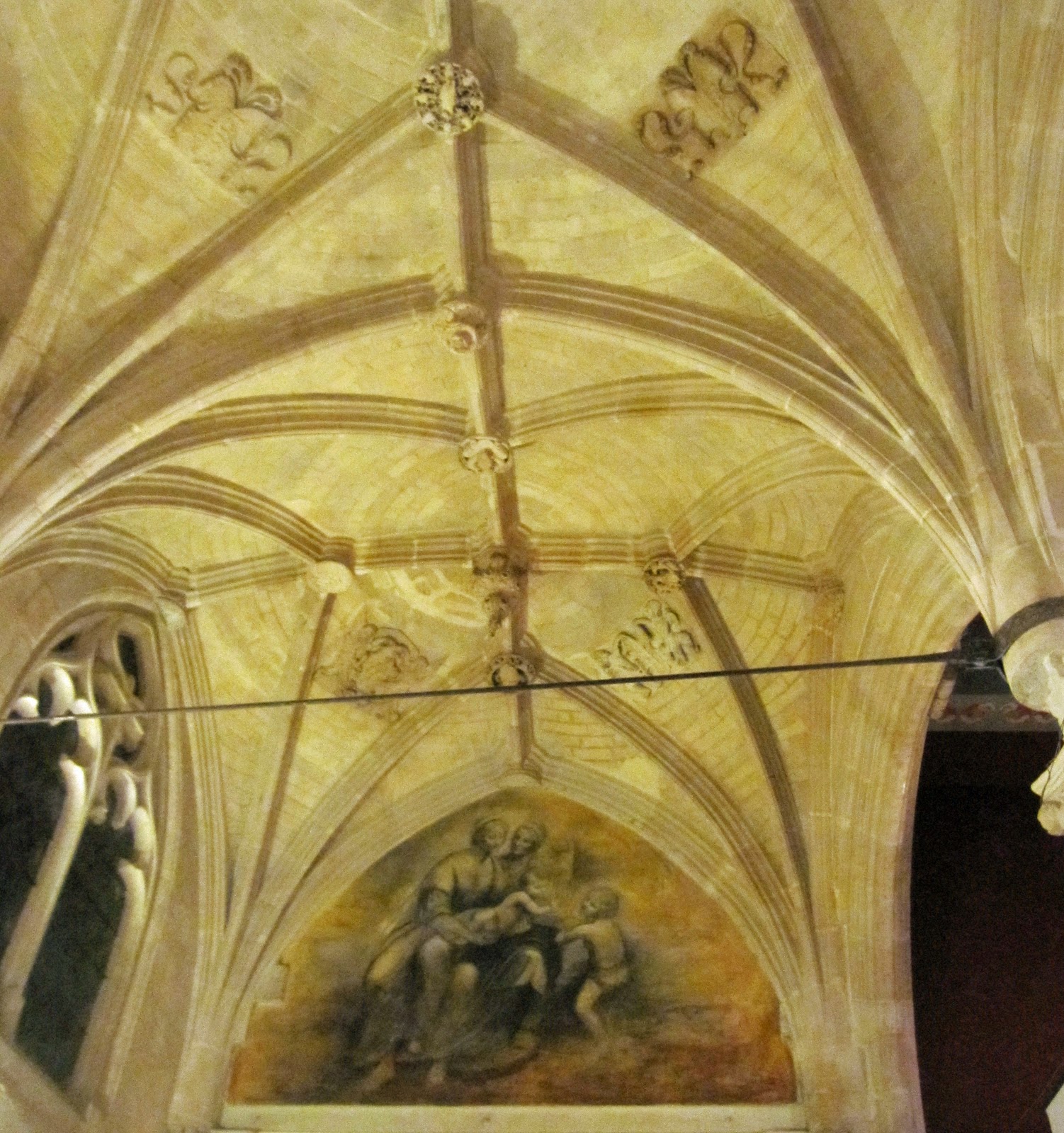The photograph captures the ornate ceiling of a chapel in a vertically rectangular frame. This full-color image, centered on the intricate architectural and artistic details of the ceiling, highlights a blend of pale yellow and white tones. The ceiling features stunning arches and support beams, with columns that extend upwards and transition into thinner, spider-like structures crisscrossing the ceiling.

At the intersection where the ceiling and wall meet, there is a prominent arch-shaped artwork. The artwork, which appears to be both painted and sculpted, presents a religious scene – several figures, including adults and children, surround a central figure, possibly Jesus, draped across their laps. The figures are depicted in a black sketch style against a dark yellow background.

Additionally, a wire runs horizontally across the center of the image, and in the lower corners, blackness frames the photograph, highlighting the central focus of the ceiling's ornate beauty.